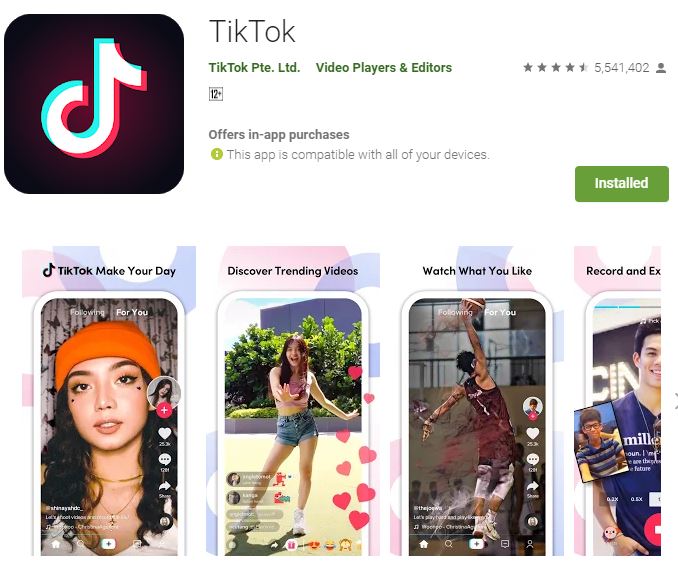This image displays the Google Play Store page for the TikTok app. Prominently featured is the TikTok logo alongside the app's name, "TikTok." The developer is tiktokpte.ltd, and it falls under the "Video Players and Editors" category. The app is rated for users aged 12 and up and supports in-app purchases. Notably, the app is shown to be compatible with all user devices. It has received 5,541,402 reviews, and the installation status indicates that it is already installed on the device. A green "Install" button is visible.

The page includes several screenshots to highlight app features. The first screenshot is titled "Make Your Day" and features a woman wearing an orange beanie, with TikTok interface elements overlaid on the screen. The second screenshot promotes discovering trending videos, showing a girl dancing outdoors accompanied by TikTok interface elements. The third screenshot, labeled "Watch What You Like," depicts a man playing basketball, again with TikTok interface elements.

The overall design of the page has a clean, white background with black text for enhanced readability. The screenshots are prominently displayed, each containing various TikTok interface icons like the like, comment, and share buttons. The layout adheres to the typical Google Play Store format, focusing on showcasing the TikTok app's features and user interface through descriptive captions and vivid visuals.